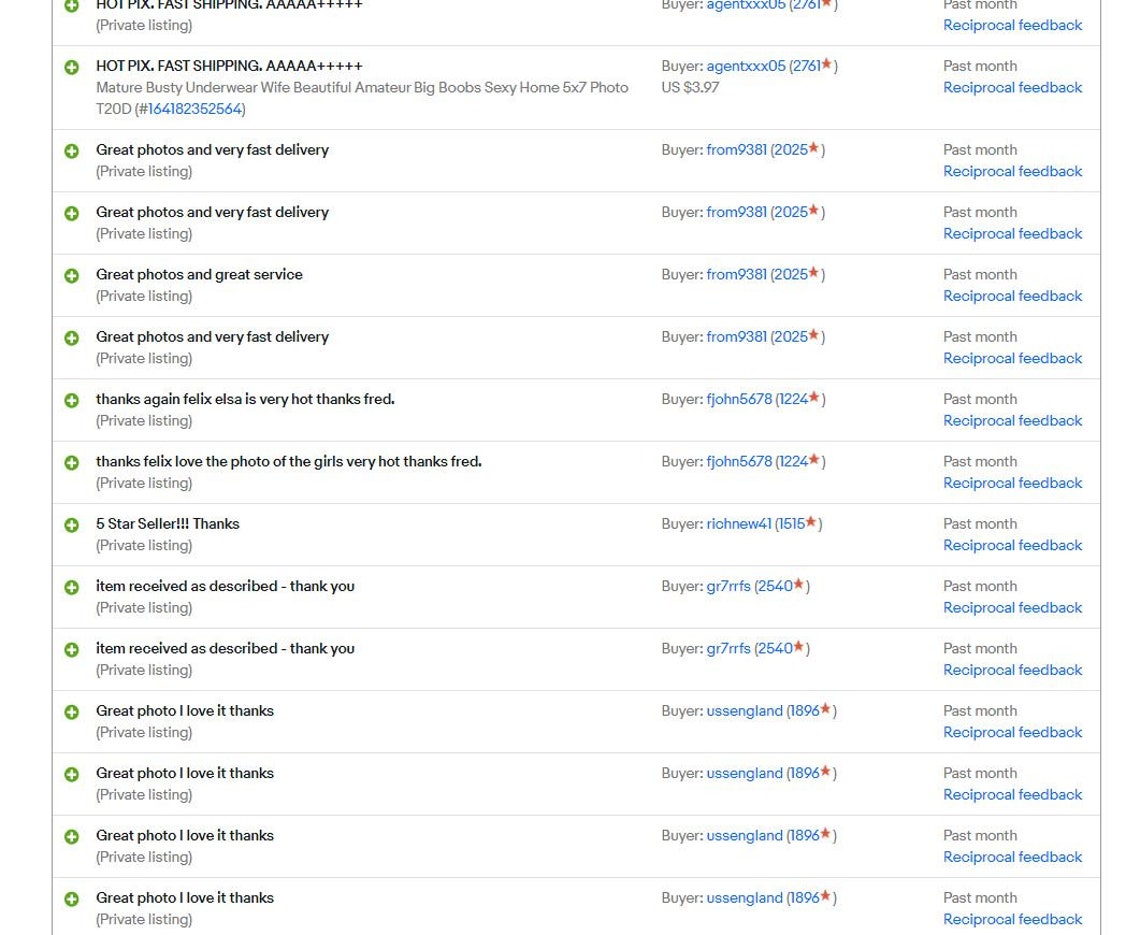This screenshot captures the reviews or feedback page from eBay, structured into three distinct columns. The left column contains the reviews and item listings, detailing the experiences and products purchased by buyers. The middle column features the buyer information, providing insights into the individuals who left the reviews. The right column is uniformly titled "Past Month Reciprocal Feedback" for every row, with the first two rows displaying different content. The page includes 15 rows, each marked with a green plus symbol, indicating positive feedback.

At the top of the page, a header reads "Hot Picks, Fast Shipping, AA, AAA, Plus, Plus, Plus, Plus, Plus," followed by the notation "Private Listing." The feedback from one specific buyer, identified as agent XXX05 (2761), is highlighted, underscoring their positive review and interaction. The layout and detailed presentation of reviews offer a clear view of the buyers' satisfaction and the seller's service quality.